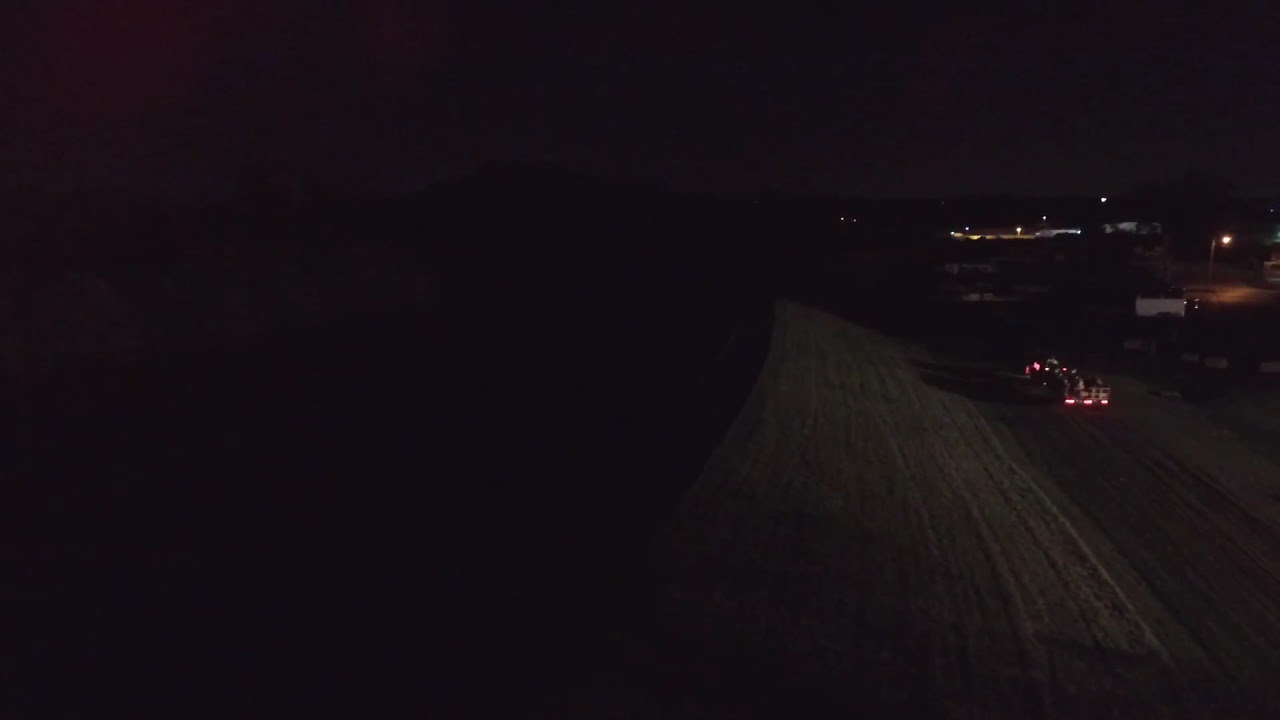This nocturnal photograph captures a very dark and shadowy scene. The image's left half is almost entirely submerged in deep blackness, rendering any details indiscernible. On the right half of the image, there is an uneven path or road, possibly composed of dirt or stones, stretching from the bottom right to about halfway up the image. Adjacent to this road, at the right side of the frame, stands a vehicle with faint red taillights, suggesting it could be a semi-truck or some form of machinery. Behind this vehicle, there are obscure shapes that hint at additional vehicles or machinery in the distance. Illuminating the scene slightly are a few street lamps positioned along the right edge, shining their light on a forlorn lot and barely touching the indistinct structures that might be buildings or houses in the far background. The sky overhead is an impenetrable dark grey, devoid of any lunar or stellar light.